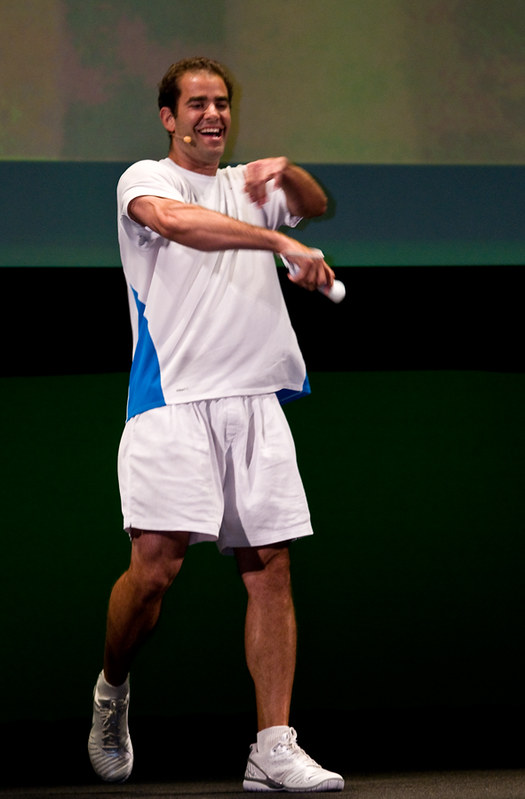The image depicts the renowned tennis player Pete Sampras mid-presentation. He's shown laughing, with a yellowish microphone attached to his right ear, extending towards his mouth. He has short brown hair, thinning at the top, and is dressed in a relaxed, athletic outfit: a white short-sleeved t-shirt with blue panels on the sides, white baggy shorts, and white athletic shoes paired with white socks. His right arm is raised, holding a white object, possibly a piece of paper, while his left arm is extended across his body in a gesturing manner. The background is primarily dark, comprising sections of black, turquoise, and lighter shades, possibly lined. Sampras appears animated and engaged, likely addressing a crowd.